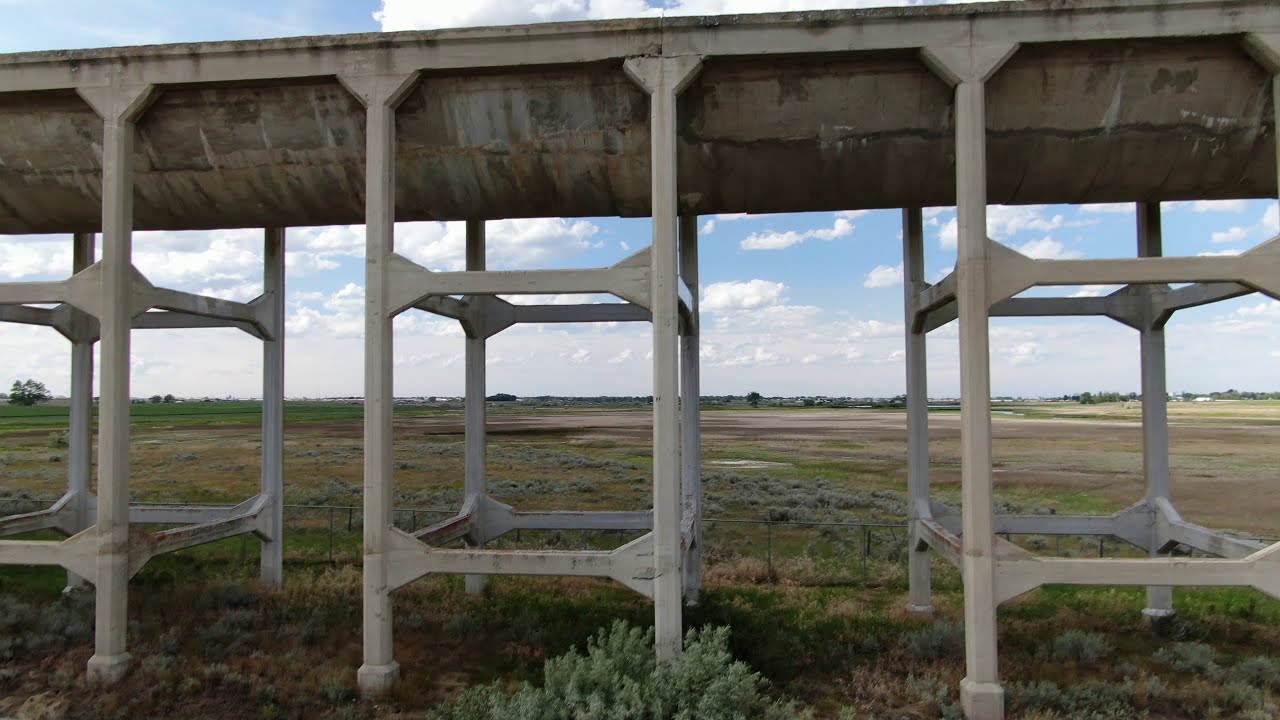This photorealistic image captures an outdoor scene featuring a large, horizontal pipeline supported above the ground by interlocked metal structures. These grey metal supports form square-shaped frameworks with horizontal and vertical components, grouped in fours—two on each side of the pipeline. The robust supports elevate the pipeline high enough that it appears a person could walk beneath it. The scene is set in a grassy field, where the grass varies between green and brown tones, indicating a mix of healthy and dry patches. Bushes and desert shrubbery are visible in the foreground, adding to the diverse vegetation.

Beyond this immediate area, a metal fence stretches across the landscape, separating the foreground from the expansive fields that blend brown dirt with green grass. The distant horizon reveals patches of darker, dry land. The sky dominates the background, filled with light blue hues and dotted by fluffy white clouds that suggest an overcast day. The sunlight is diffused, creating a soft, even light across the scene. Trees and possibly residential areas are faintly visible in the far distance, blending into the vast, open environment. Overall, the image evokes a sense of a calm, rural landscape, possibly located in the western United States, with a distinct structure as its focal point.